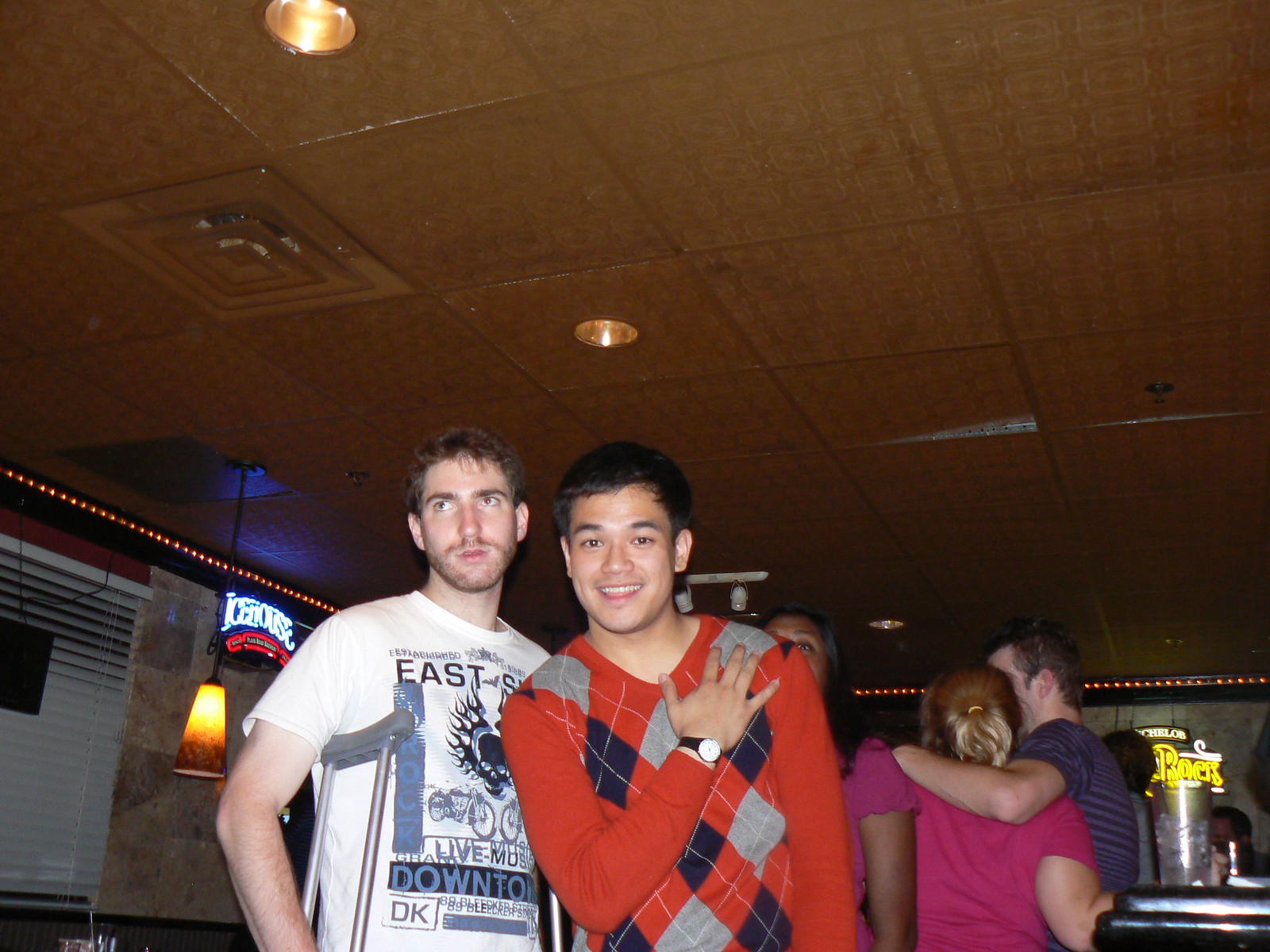The photo is taken inside a bar with a light brown tile ceiling, a vent, and ceiling lights. Dominating the center of the image are two young men. The first is an Asian man with black hair, dark eyes, and a watch, smiling at the camera with his hand near his heart. He wears an Argyle sweater in orange, red, blue, and gray. To his left stands a white man with medium-length black hair, a beard, and a mustache. He is wearing a graphic t-shirt and has crutches under both arms. In the background, a man with his arm around a woman in a pink shirt can be seen. The bar area is visible on the right, featuring a neon sign against a stone wall. White blinds cover a window on the left side of the image. The overall scene captures a cozy, communal atmosphere with intricate details and interactions among the people.